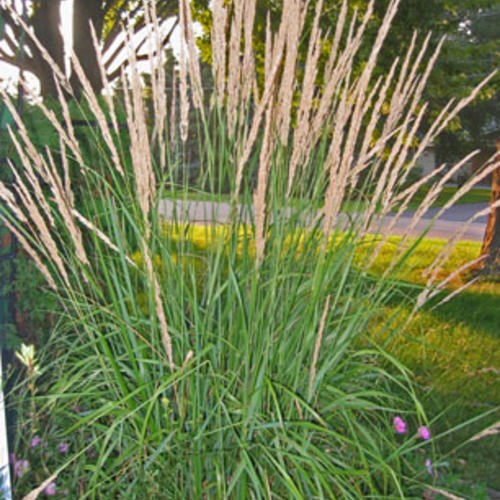In this square, daytime photograph taken with an auto setting, we see a vibrant outdoor scene dominated by a sawgrass plant, characterized by its tall, thin green blades and light brown seed spikes that resemble wheat stalks. The grass area is extensive and wide, with long green grass interspersed with light brown flowers. In the foreground, there are also small purple and pink wildflowers adding a splash of color. The sunlight throws a warm late afternoon glow over the scene, casting shadows on the ground.

In the middle distance, a gray road or pathway cuts through the grassy expanse. This pathway is bordered by verdant green trees, and on the upper left, there's a tree trunk that splits into two, with a white sky creating a backdrop. Further in the background, partially obscured, is a house or building, possibly a brown ranch-style home or a white garage, contributing to the depth of the image. Overall, the photograph captures a richly textured and sunlit natural landscape.